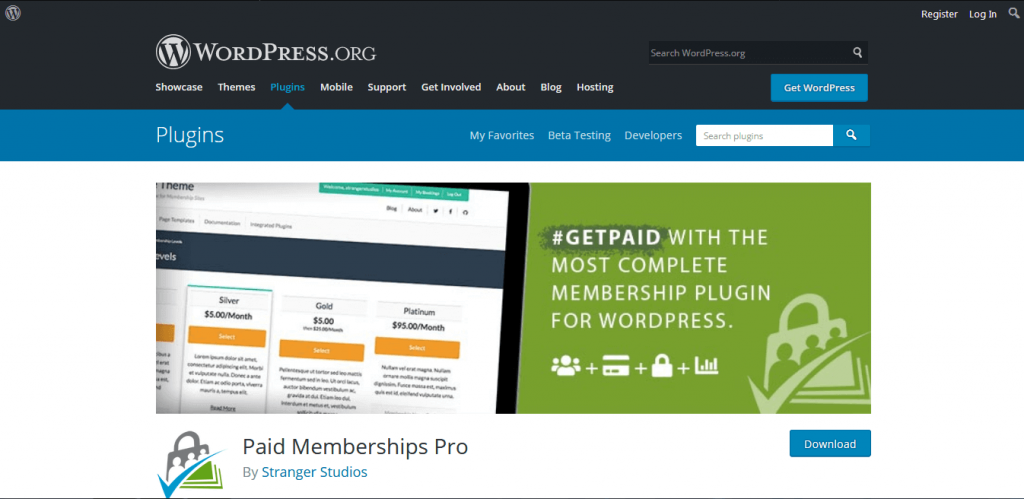This screenshot from the website WordPress.org highlights the platform's focus on various plugins, particularly those related to accessing exclusive content. The user is exploring paid membership options for pro users, indicated by a prominent green checkmark over a locked icon, serving as the principal logo for this feature. The site offers a detailed overview of subscription pricing and showcases additional tools such as blog posts and mobile support sections under specific headings and themes.